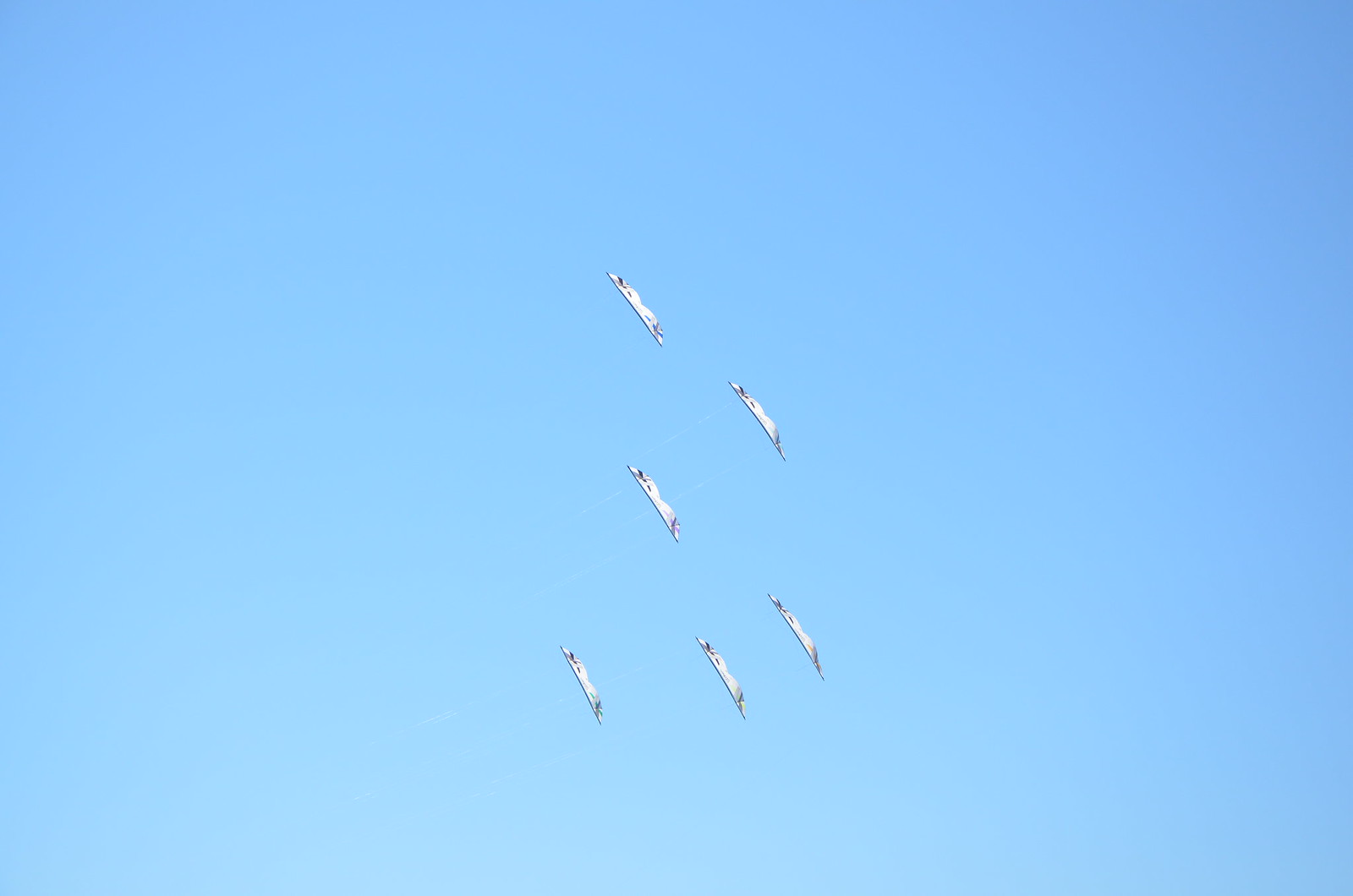This is an outdoor photograph taken on a clear day, showcasing a vast expanse of bright blue sky without any clouds. Positioned in the middle of this sky are six distinct, identical objects that resemble small, boomerang-shaped airplanes. They are aligned in a formation, but instead of flying level, they appear to be turned at angles, possibly at 60 or 90 degrees, which reveals their thin, flat profiles. Though there are no visible strings, contrails can be seen trailing from these objects, suggesting movement and supporting their identification as aircraft. The image is simple, with nothing else in the sky to distract from these six intriguingly angled flying objects.